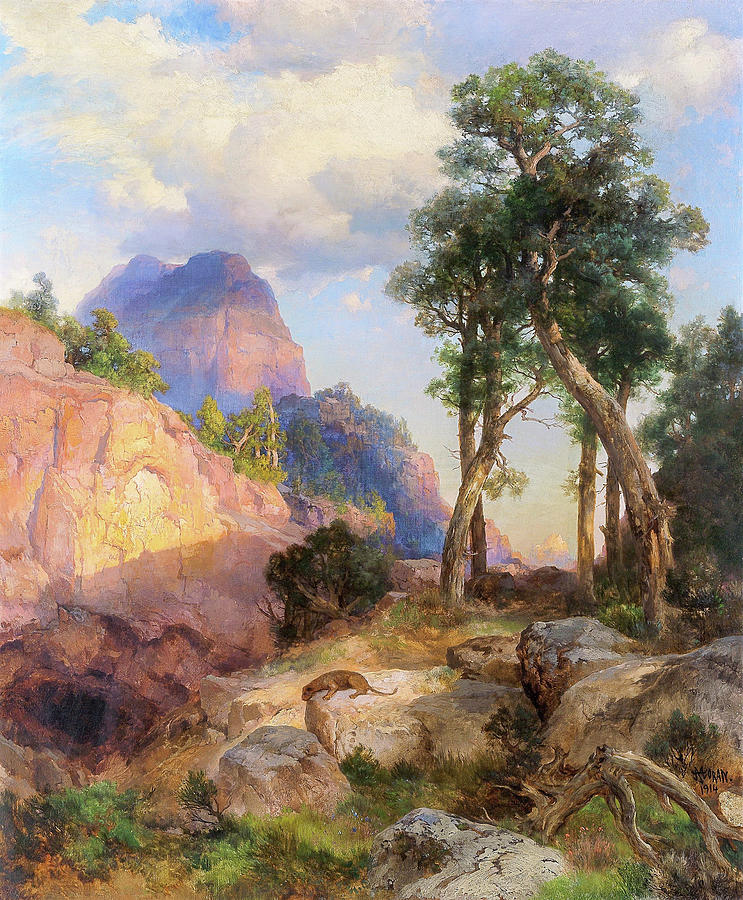The painting, rendered in watercolor and dated 1914, captures a serene outdoor landscape with meticulous attention to detail. The scene is dominated by a rugged terrain of large boulders and rocks interspersed with green grasses and shrubs, leading up a hill. At the center of the composition, illuminated by sunlight, is an ambiguous animal, possibly a mountain lion or a dog, laying on a central boulder and gazing downwards. The animal is characterized by a low, long back, a thin tail, and large, hunched hind legs, facing towards the left-hand side.

To the left, the painting features steep, imposing cliffs, extending upwards to meet a bright blue sky filled with large, billowing clouds. At the midline on the left-hand side, five tall trees rise from the ground, their branches prominently stretching out at the top. The rightmost tree exhibits a notable leftward curve at its base.

Further down the left side at the base of the hill, a dark cave entrance adds a sense of mystery. Behind the hill, formidable mountain ranges frame the background. The lower right-hand corner of the painting bears the artist's signature, resembling "M crossed with an A, O-R-A-N." The scene is suffused with vibrant, almost idyllic light, reminiscent of the colors seen in works by Maxfield Parrish.